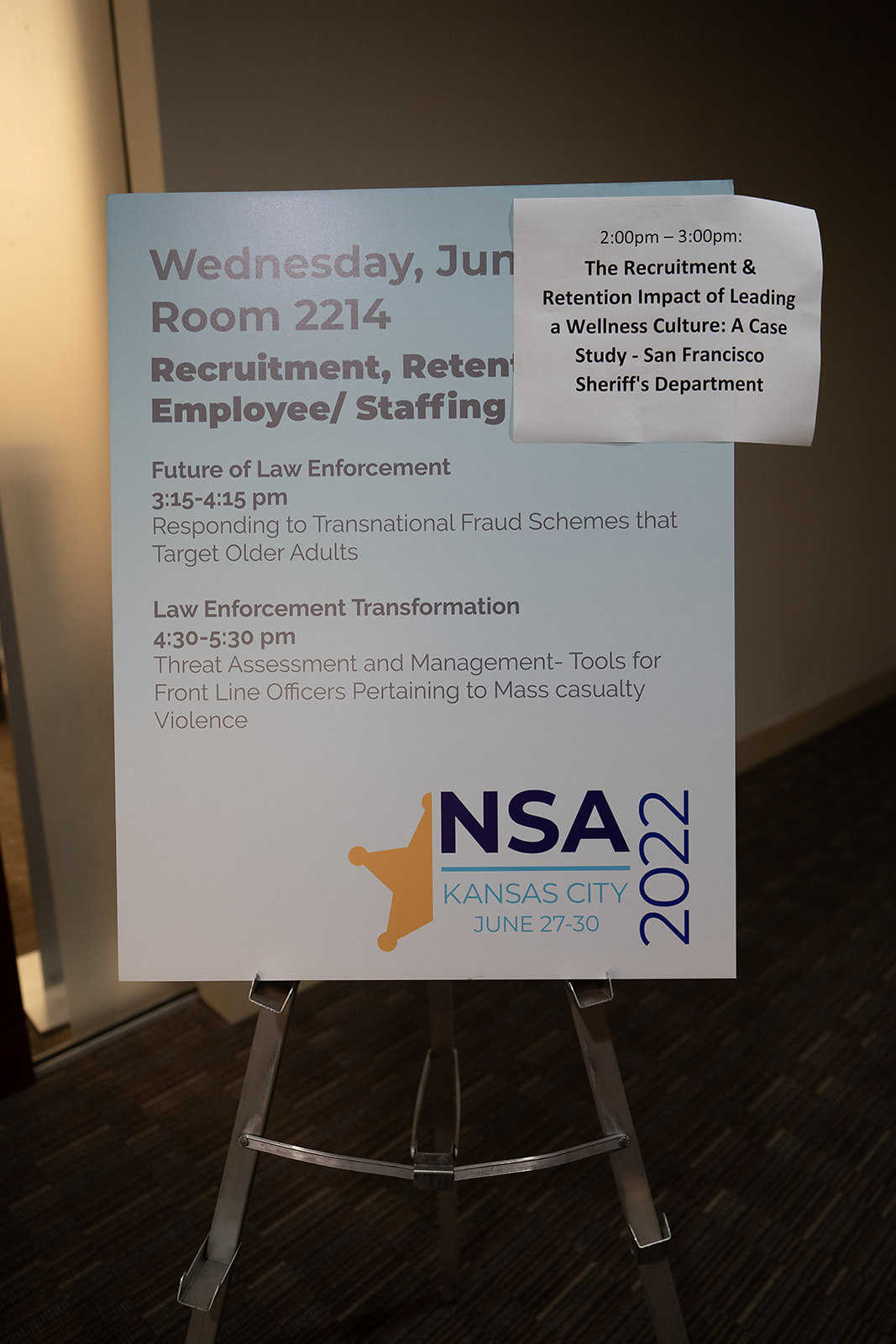The image depicts a detailed schedule poster for a law enforcement conference, displayed on a metal stand in what appears to be a showroom. The main poster lists event details under the heading "Wednesday, June" before being cut off. The scheduled events are held in room 2214 and include sessions on recruitment, retention, and employee staffing. Specifically, from 3:15 to 4:15 PM, there is a session titled "Future of Law Enforcement" focused on responding to transnational fraud schemes that target older adults. Following this, from 4:30 to 5:30 PM, another session titled "Law Enforcement Transformation" will cover threat assessment and management tools for frontline officers dealing with mass casualty violence. Additionally, a small white piece of paper affixed to the top right of the main sign amends the schedule with an earlier session from 2:00 to 3:00 PM on "The Recruitment and Retention Impact of Leading a Wellness Culture: A Case Study by the San Francisco Sheriff’s Department." At the bottom right of the poster, the logo features the NSA in dark blue colors with "Kansas City, June 27th to 30th" beneath it, and "2022" is printed vertically alongside the logo.